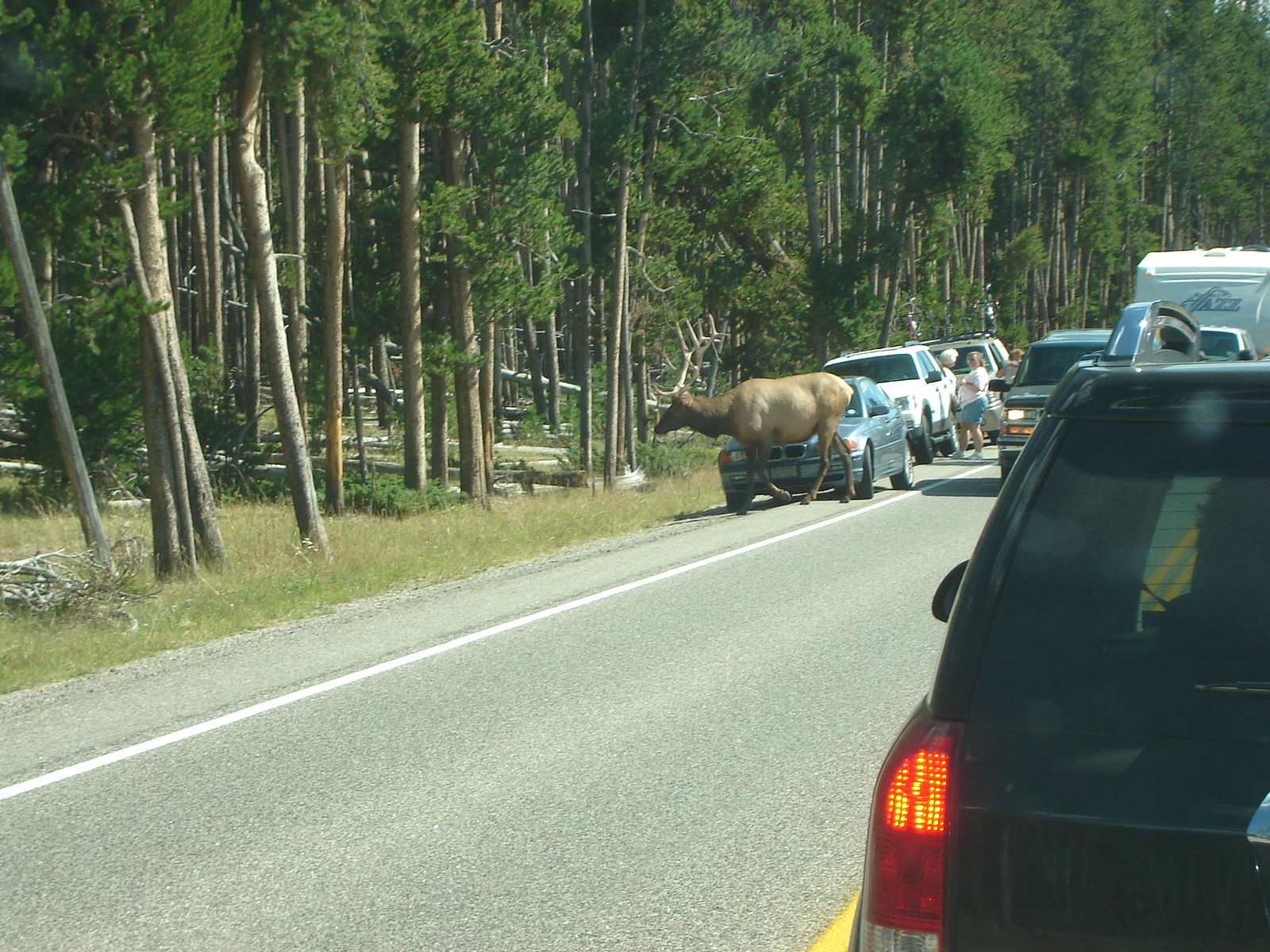The image captures a large brown moose crossing a busy road, highlighting its impressive size in comparison to the surrounding vehicles. The moose, particularly dark brown around its head and neck, sports imposing antlers and is positioned near a light blue car. The roadway is lined with parked vehicles and active traffic, including northbound and southbound lanes. On the left side of the image, a dense forest with tall, leafy trees creates a natural backdrop. To the right, a black SUV is seen, emphasizing the contrast between the natural wilderness and bustling roadway.